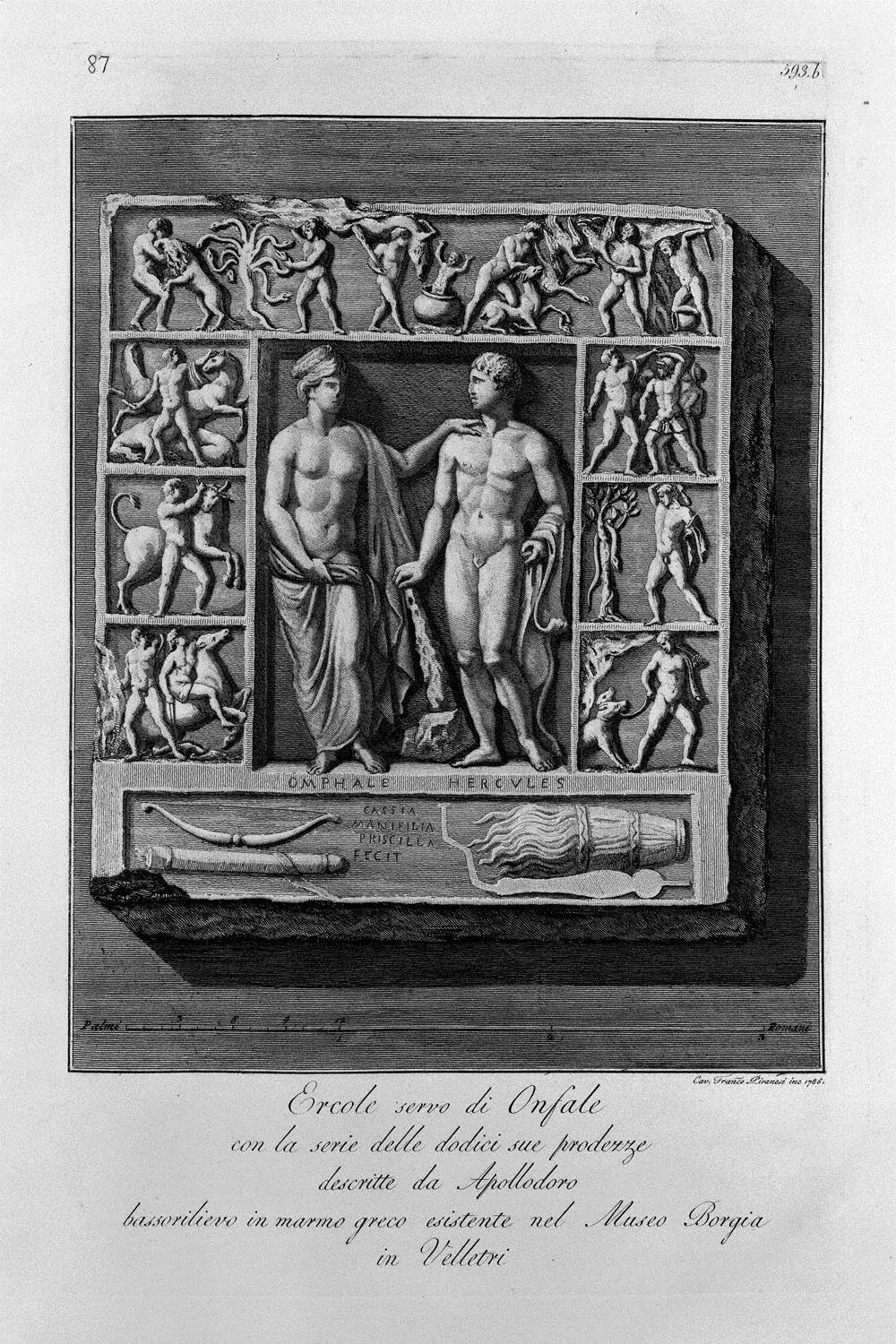The image depicts a detailed, pen-and-ink artwork designed to resemble a classical piece of art with predominant shades of gray. Structured in a poster-like format, it features several panels resembling scenes you might find in a stained glass window or on a series of shelves. At the bottom of the artwork, there's a lengthy inscription written in what appears to be Latin or possibly Greek: "Ercole Servo di Onfale conta serie delle dodici sue Prodenze," followed by additional smaller text in the same foreign language.

The central panel displays two men in classical attire, one possibly wearing a Roman toga while the other may be partially nude or in a robe. Surrounding the central figures are six smaller boxes, framing the image on the left, right, and top. Each smaller panel illustrates various activities: one shows a man with an animal, and another depicts two individuals alongside an animal. There is also a panel with a figure wearing a hat adorned with leaves. At the top, a panel combines multiple dynamic scenes, including a man battling an animal and another figure fighting with what seems to be a tree.

Overall, the artwork intricately combines elements of classical representation with a hint of narrative storytelling through its sequential panels and detailed inscription.